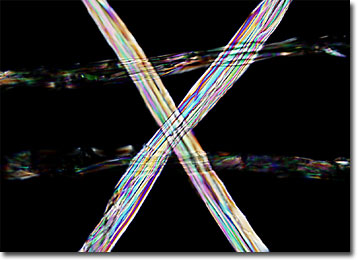This horizontally aligned rectangular painting features a solid black background with two smudged horizontal lines extending across it, roughly near the top third and bottom third. These horizontal streaks blend together in various shades of black, gray, and white. Dominating the center of the artwork is a prominent X shape, with each arm of the X stretching from corner to corner. The X is filled with an array of colors, including blue, purple, white, black, orange, red, gold, green, and brown, as well as darker shades of purple and lighter shades of blue. The colors within the X are densely packed and noticeably vibrant, contrasting with the more muted horizontal streaks. The painting is a striking composition of vivid intersecting lines against a dark, minimalistic backdrop.